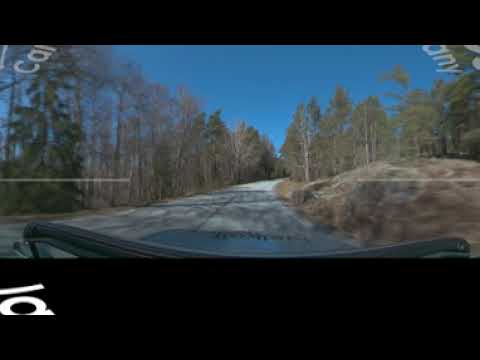This daytime image, likely captured by a dashboard camera possibly mounted on a Jeep, showcases a scenic rural road winding slightly to the right. The bottom portion of the picture is black with fragmentary white lettering, including characters resembling "L" and "A" on the left and "C-A-O" and "A-N-Y" on the right. The hood of the vehicle is visible just below the windshield. On either side of the gray-paved road, rows of trees create a serene atmosphere, with many bare branches suggesting a fall setting. On the right, brown foliage and several trees extend into the backdrop, and a large green pine tree stands prominently on the left. The background reveals light blue skies, free of any clouds, capped by rolling hills and trees that add to the tranquil rural charm.